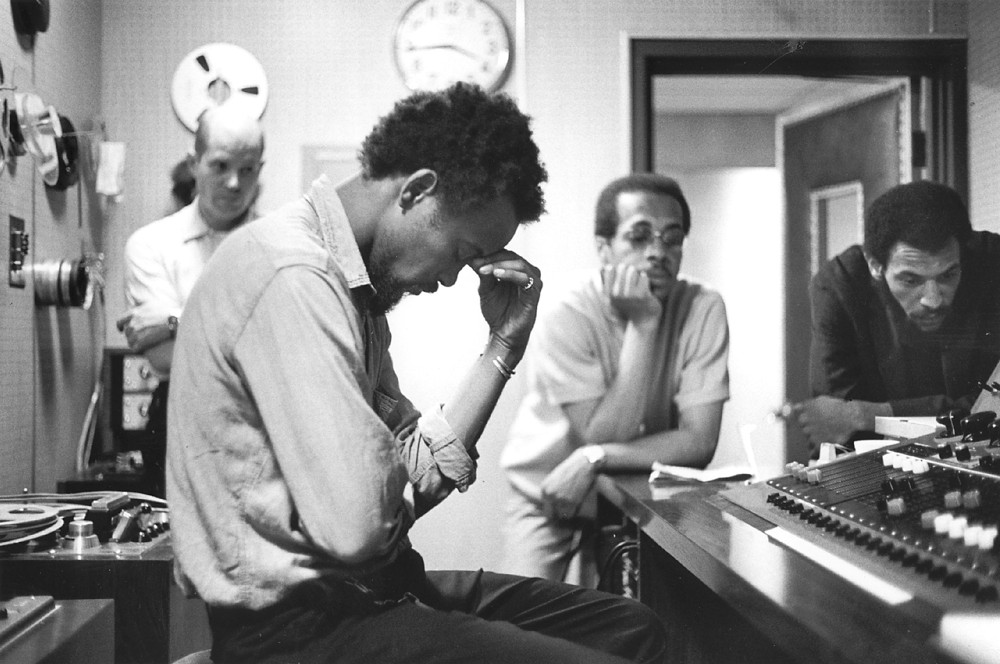The black-and-white image captures a tense moment in a recording studio, where four men are deeply engrossed in their work. The primary focus is on a young African-American male seated in the foreground, his body turned towards the right, with his head resting on his left hand, exuding an air of deep contemplation or disappointment. He is dressed in a long-sleeve collared shirt and trousers, facing a control board possibly scrutinizing a recording or deliberating a critical situation. Beside him, to the right, two more young African-American males are leaning over the control board. The one in the middle, adorned with glasses, a tan shirt, and a shiny watch, mirrors the serious demeanor, his head resting in the palm of his right hand. Next to him, another young man in a dark long-sleeve shirt leans in with both elbows on the table, focused intently ahead. In the background, a white, bald male stands slightly removed, appearing worried yet attentive, with his gaze fixed on the control board. The room is filled with various recording equipment, including a small turntable on the bottom left and some gadgets on the wall. A clock on the back wall marks the time at 3:44, encapsulating the moment of collective anticipation or problem-solving.